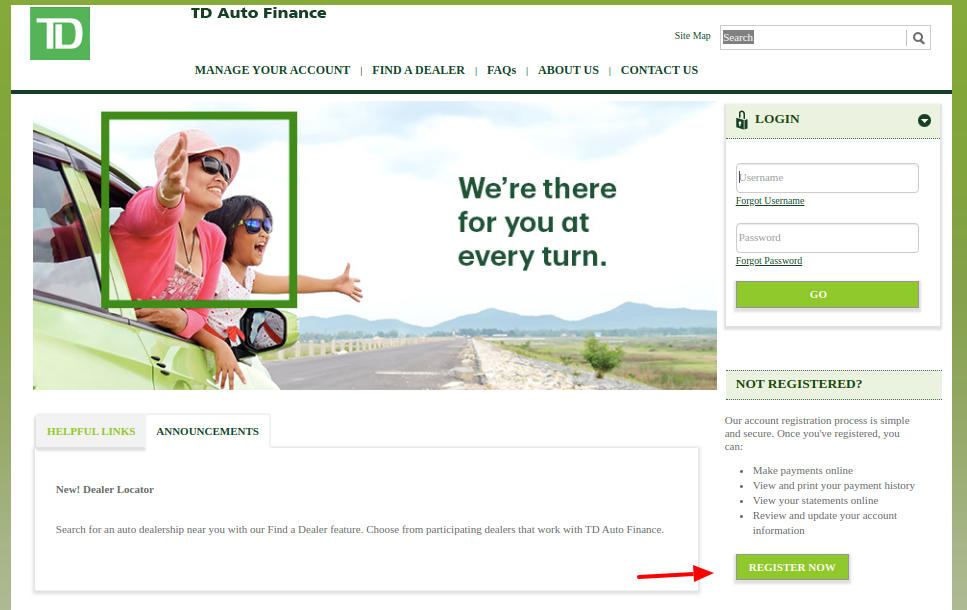The image is a screenshot of the TD Auto Finance website. The top of the page features the TD Auto Finance logo, with navigation options including "Manage Account," "Find a Dealer," "FAQs," "About Us," and "Contact Us." Below the navigation bar, a large featured image shows two people hanging out of a car with their arms outstretched, conveying a sense of freedom and joy. Accompanying this image, there is a motivational slogan on the left that reads, "We're there for you at every turn." To the right of the image is the login section, which includes a "Username" input box with an adjacent "Forgot Username" link, and a "Password" input box with an adjacent "Forgot Password" link. Below these fields is a "Go" button for submitting login information.